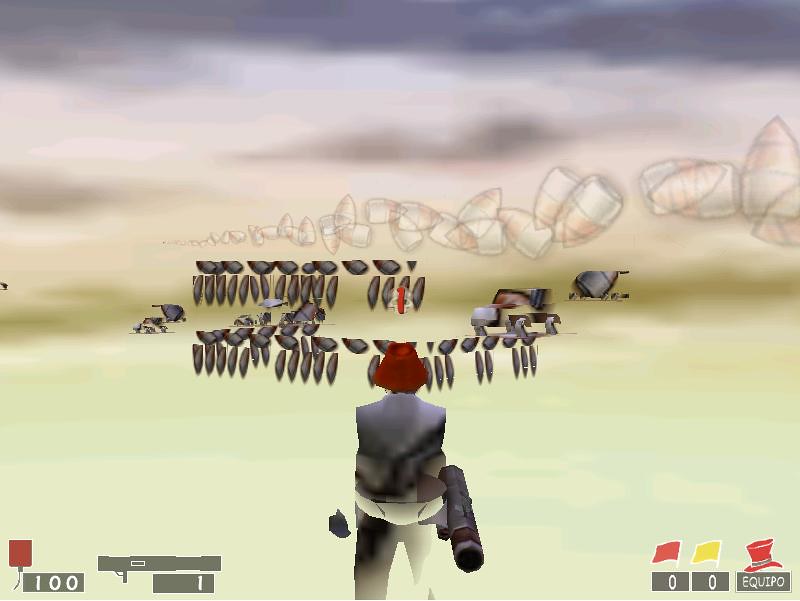In this video game screenshot, the central figure is a player-character situated in the middle of the frame, holding what appears to be a gun or cannon in their right hand. The character is facing away from the viewer, gazing into the distance. The terrain around them is stark and desolate, characterized by a white, barren ground. Scattered across the landscape in the distance are several oval-shaped objects, gray and black in color, adding to the eerie atmosphere. Additionally, various fragments of what seem to be parts of a rocket ship are strewn about the area. In the bottom right corner, a collection of red and yellow flags is visible, accompanied by a red hat, further adding to the scene's mysterious and forlorn setting.